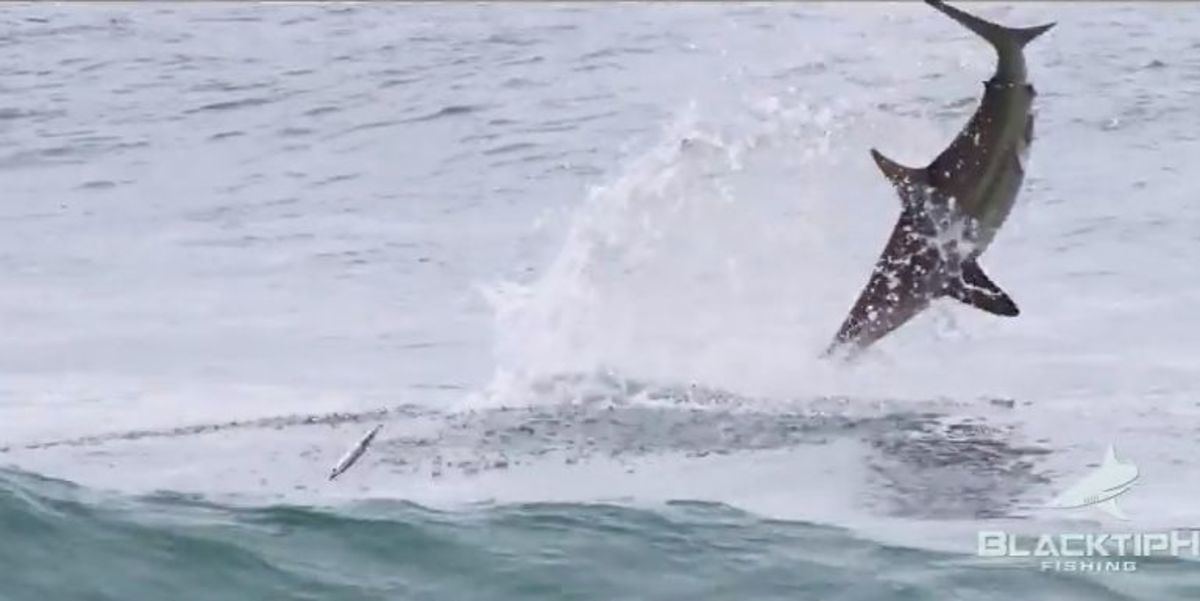A dynamic photograph captures an intense marine moment at sea, featuring what appears to be a large marlin or shark, dark gray in color, diving back into the water mid-air, with its glossy body arching and tail almost vertical near the top right. Surrounding the central figure, a cascade of water is suspended in midair, adding drama to the scene. To the bottom left, a smaller fish can be seen leaping out of the bluish-green, slightly gray-tinged water, creating a contrast in scale and motion. The water itself displays a range of motions, with small ripples in the background and progressively larger waves in the foreground. Completing the scene, the bottom right corner features a logo of a shark silhouette in off-green, accompanied by the text "Black Tip Fishing."